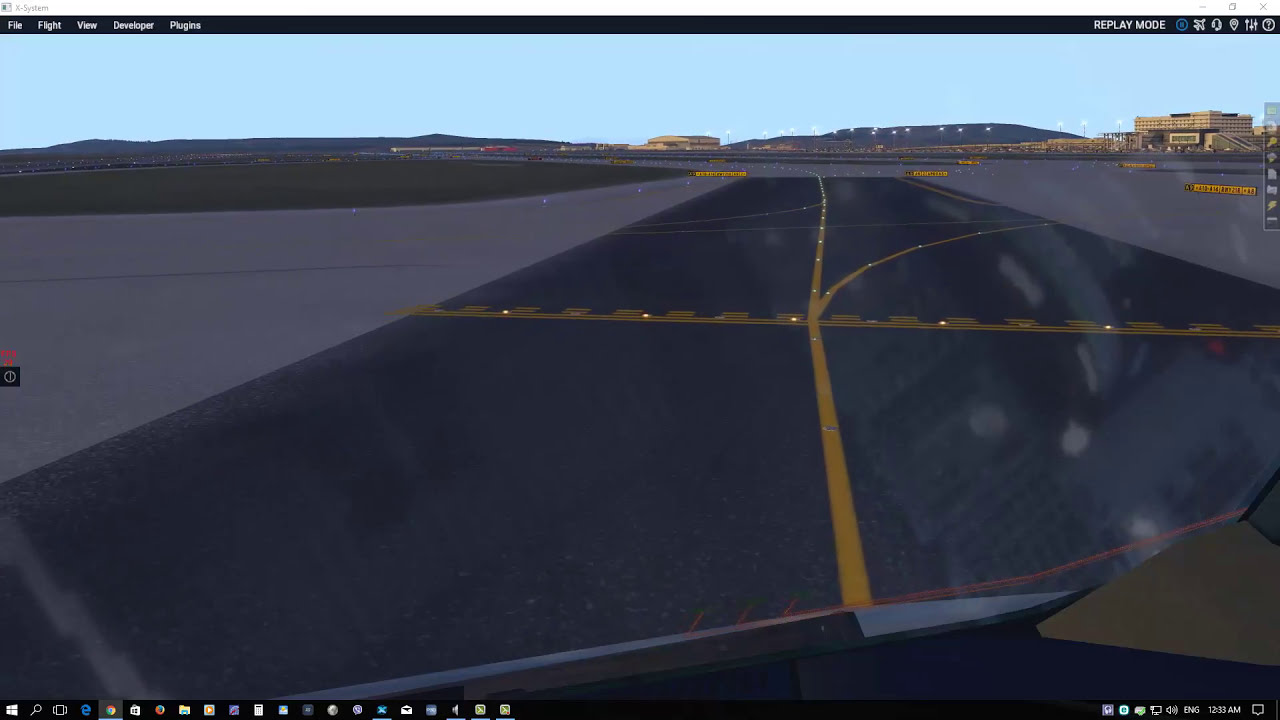The image is a horizontal rectangular screenshot of a flight simulation video game displayed on a Windows computer screen. At the top of the screen, a black bar carries the text "Replay Mode" on the right side and includes an 'X' to exit out. The menu bar beneath it lists the tabs as File, Flight, View, Developer, and Plugins. The bottom Windows taskbar shows various icons, including Internet Explorer, the Windows icon, volume control, and the time, indicated as 12:33 AM.

The scene captured in the image appears to be from inside the cockpit of an airplane, overlooking a daytime airport runway. The foreground shows a straight stretch of tarmac with a yellow line running down its center and intersecting dashed lines, resembling taxiway markings more than a racetrack. The environment is a 3D simulation featuring an airport hangar, a long expanse of airport pavement and runway, and a distant mountain range under a light blue sky. The background includes various buildings and possibly an airport hangar illuminated by lights. The overall setting is detailed with clear distinctions between the runway and surrounding airport structures against a bright, expansive sky.